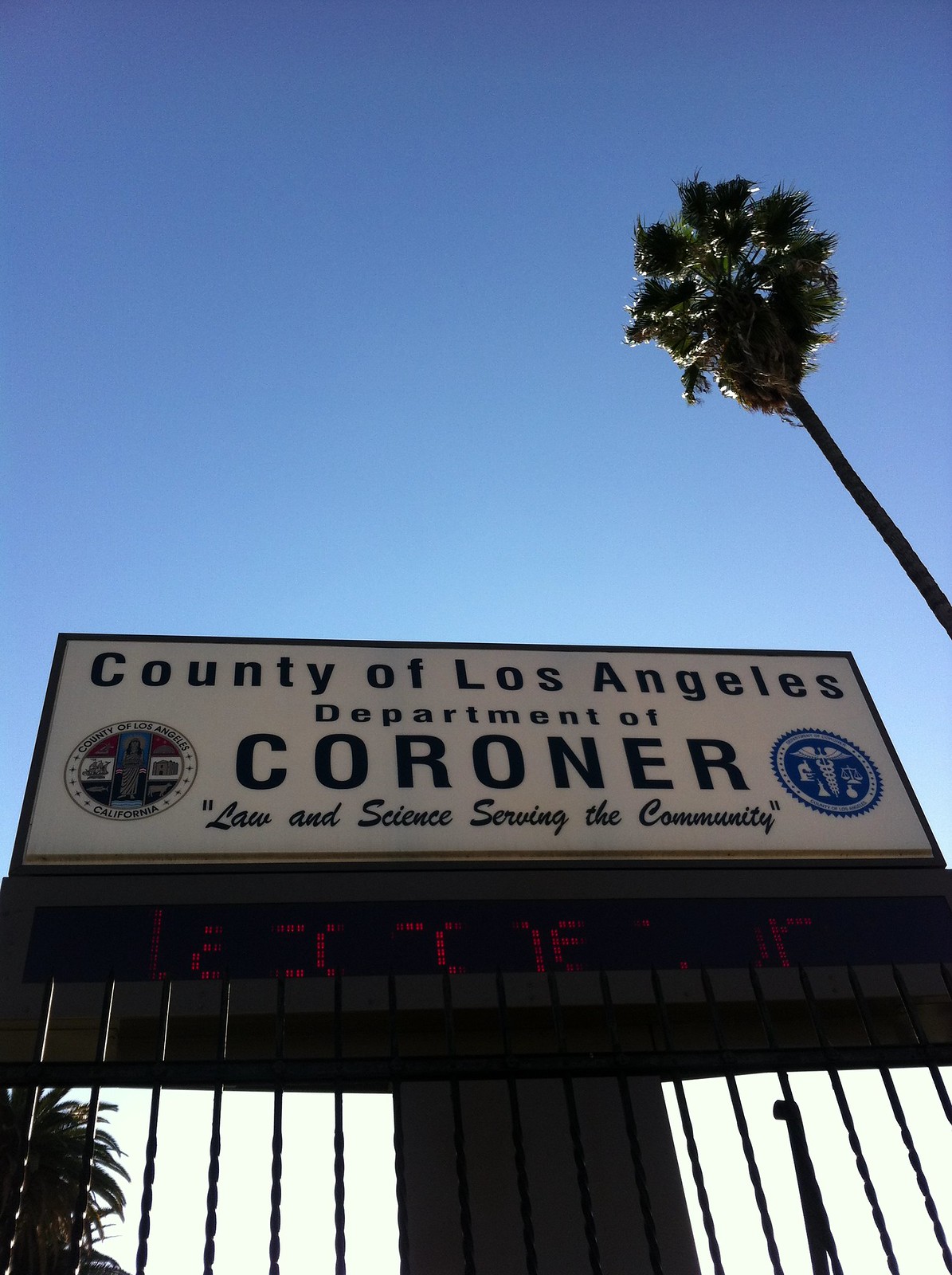This captivating image captures a sign for the County of Los Angeles Department of Coroner. The photo, taken from a ground-level perspective looking up, prominently features the sign centered against a vivid blue sky. The sign itself is a white rectangle with a thin black border, displaying the text "County of Los Angeles Department of Coroner" in black. In a handwritten script, the phrase "Law and Science Serving the Community" is quoted beneath. Flanking the word "Coroner," there are two logos: on the left, the official County of Los Angeles logo, and on the right, a medical emblem with wings and a spiral design. Below the main sign is a digital screen with red illuminated text that is difficult to read in this image. The scene also includes a gate and several black bars at the base of the sign, possibly part of a fence. Notably, a single palm tree peeks into the frame from the right, adding a touch of nature to this otherwise official setting.